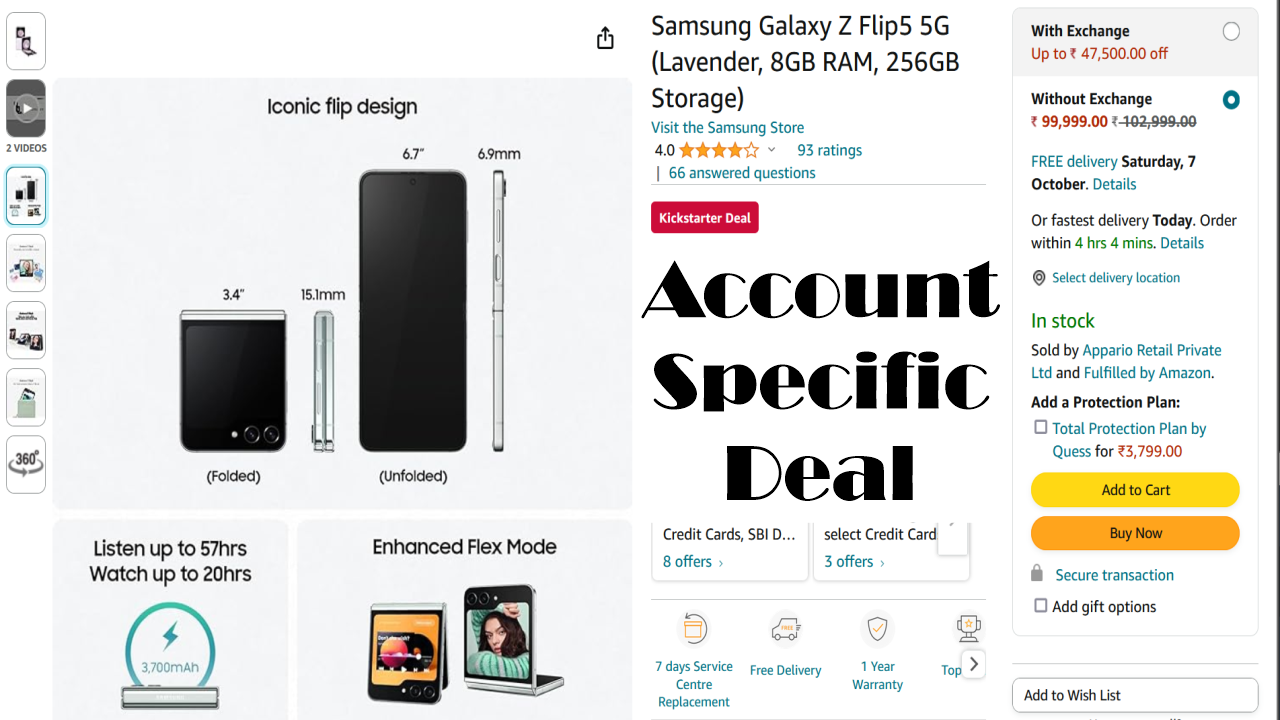This image showcases an Amazon product page for a mobile phone. The featured product is a "Samsung Galaxy Z Flip 5," a 5G phone available in Lavender color with 8GB of RAM and 256GB of storage. On the left side of the screen, there is a vertical strip displaying different smaller images of the phone, showcasing various angles and features. The highlighted section shows the phone folded, a side view, the phone unfolded, and another side view.

Below these images, the description notes: "Listen up to 57 hours, watch up to 20 hours," and there's an illustration under this text. Adjacent to this, the "Enhanced Flex Mode" feature is highlighted with a visual of the phone folded, displaying different images on its screens.

In the middle of the right-hand side, prominently displayed in large font, is "Account Specific Deal," followed by details regarding credit card offers such as "Credit cards, SBID, eight offers, select credit card, three offers."

Continuing down the right side, another menu presents additional options and information, indicating it's an Amazon webpage. Details include: "With exchange up to 47,500 off," "Without exchange 99,999," and "Free delivery Saturday, 7th October." There are also delivery options mentioned: "Details or fastest delivery today. Order within four hours and four minutes. Select delivery location."

The product is listed as "In stock," sold by "Apario Retail Private Limited" and fulfilled by Amazon. Below this, you find the "Add to Cart" and "Buy Now" buttons, secure transaction options, and an "Add gift options" link.